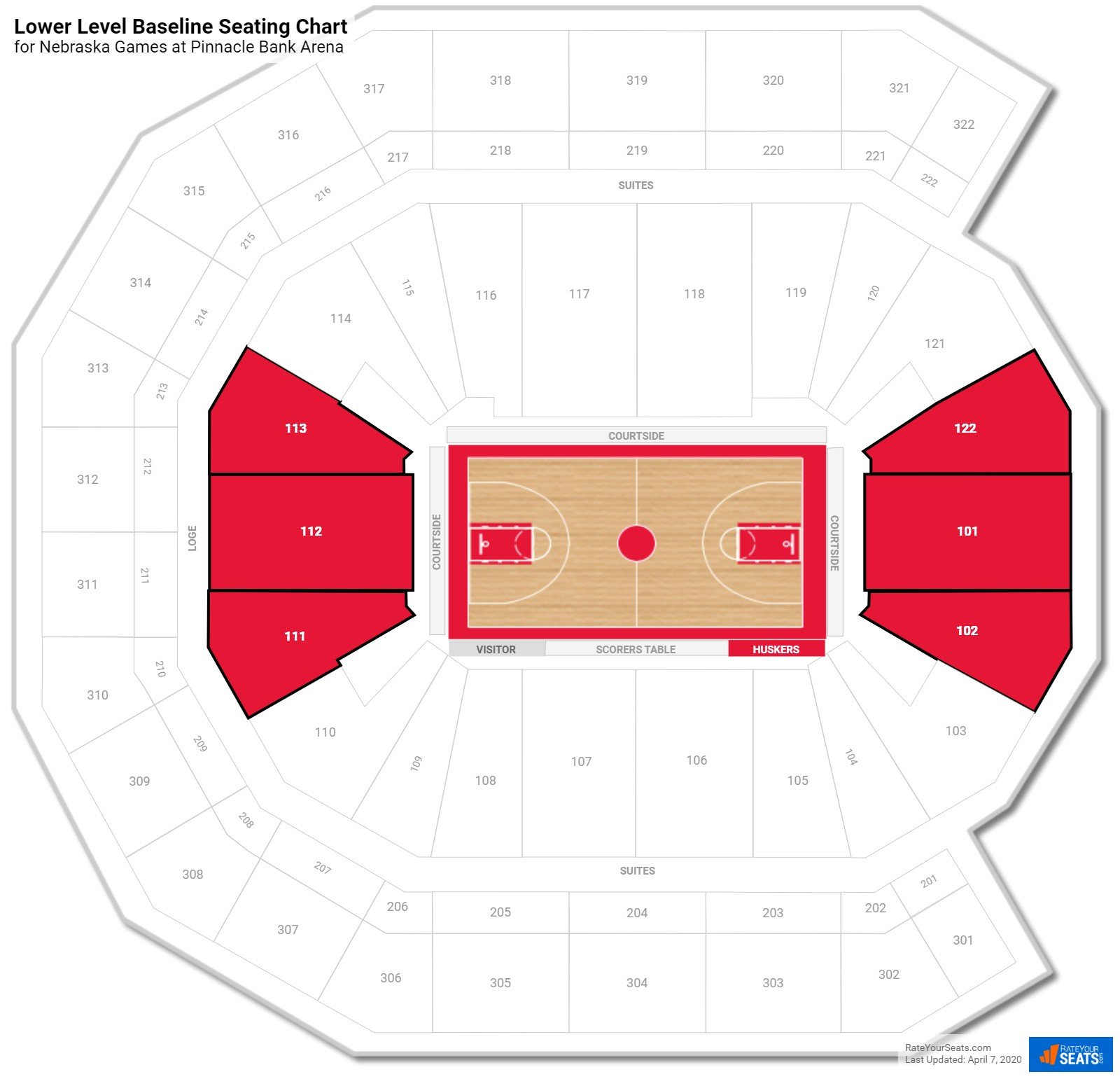This detailed aerial illustration image provides a comprehensive view of Pinnacle Bank Arena, specifically focusing on the lower level baseline seating chart for Nebraska games. The image has a clean white background, enhancing the clarity of the intricately designed stadium layout. 

In the upper left-hand corner, black text denotes "Lower Level Baseline Seating Chart for Nebraska Games at Pinnacle Bank Arena." Dominating the center is the detailed illustration of the arena, where the basketball court stands out with its brown and red flooring, complemented by white court markings.

To the left and right of the central court, sections 113, 112, and 111 on the left, and sections 122, 101, and 102 on the right are prominently highlighted with black outlines and shaded in red for easy identification.

All other sections are meticulously marked with light gray borders and numbered in the center, ensuring thorough navigability. The entire arena illustration is encased in a medium gray thick border, adding definition to the overall layout.

In the lower right-hand corner, the logo "rateyourseats.com" is displayed, along with a note indicating the last update on April 7, 2020. Adjacent to this is a blue button icon encouraging viewers to "Rate Your Seats."

This thoughtful and detailed caption ensures that the viewer gets a complete understanding of the seating arrangement and layout of Pinnacle Bank Arena as depicted in the illustration.